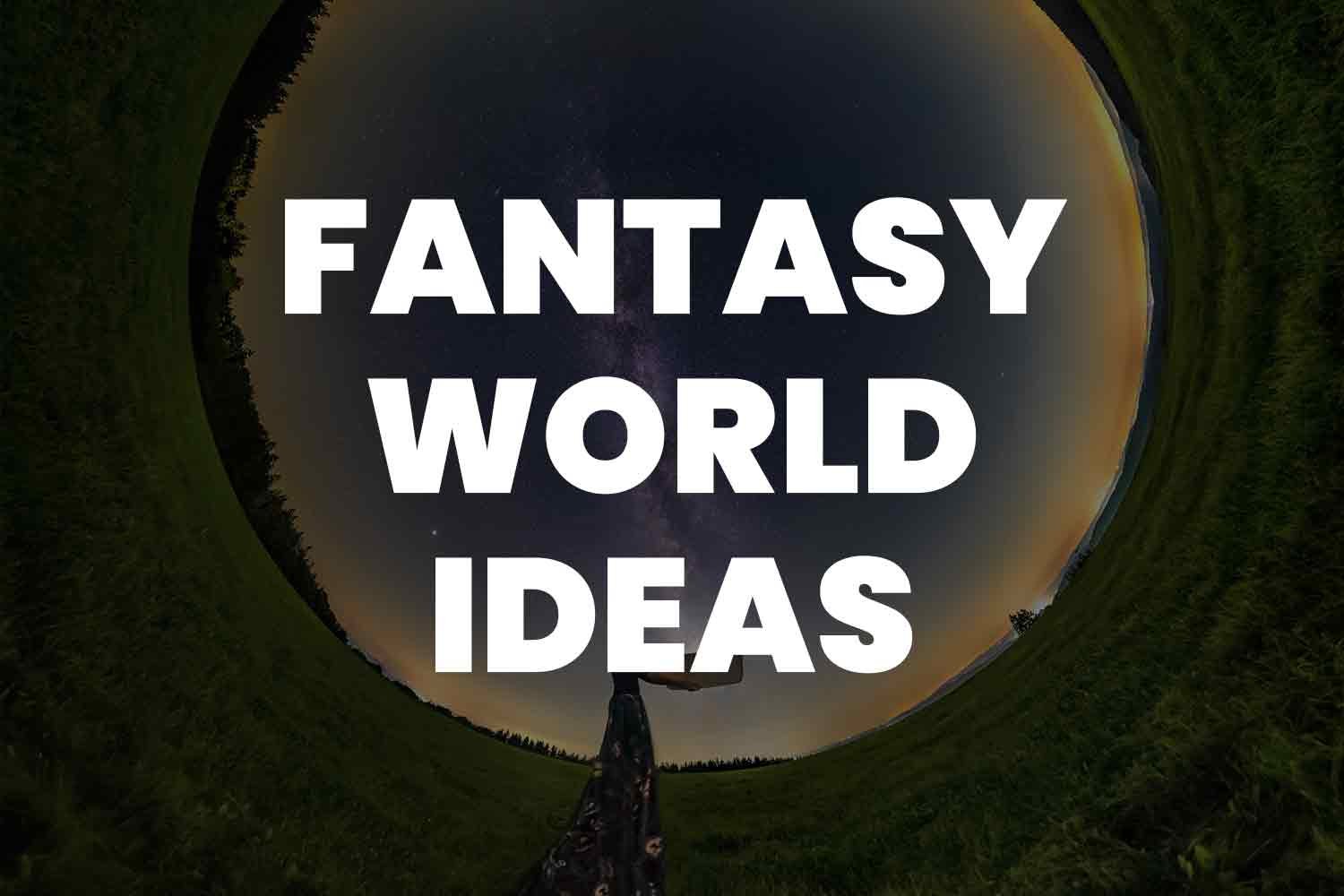The digitally altered image features a surreal night-time landscape. The scene is presented in a circular format, almost as if one is peering through a large, dark tunnel. The landscape, covered in grass and dotted with trees, wraps continuously around the edges, creating a ring. The night sky within the ring graduates to a yellowish hue, hinting at the remnants of a sunset. Prominently displayed across the center is bold, white text reading "Fantasy World Ideas," obscuring parts of the image. Near the bottom center, partially hidden by the text, stands a figure. The visible portion of this person reveals legs clad in a dark blue dress adorned with a floral pattern. Additional elements, such as a couple of buildings, contribute to the intricate circular design of the digitally manipulated scene.